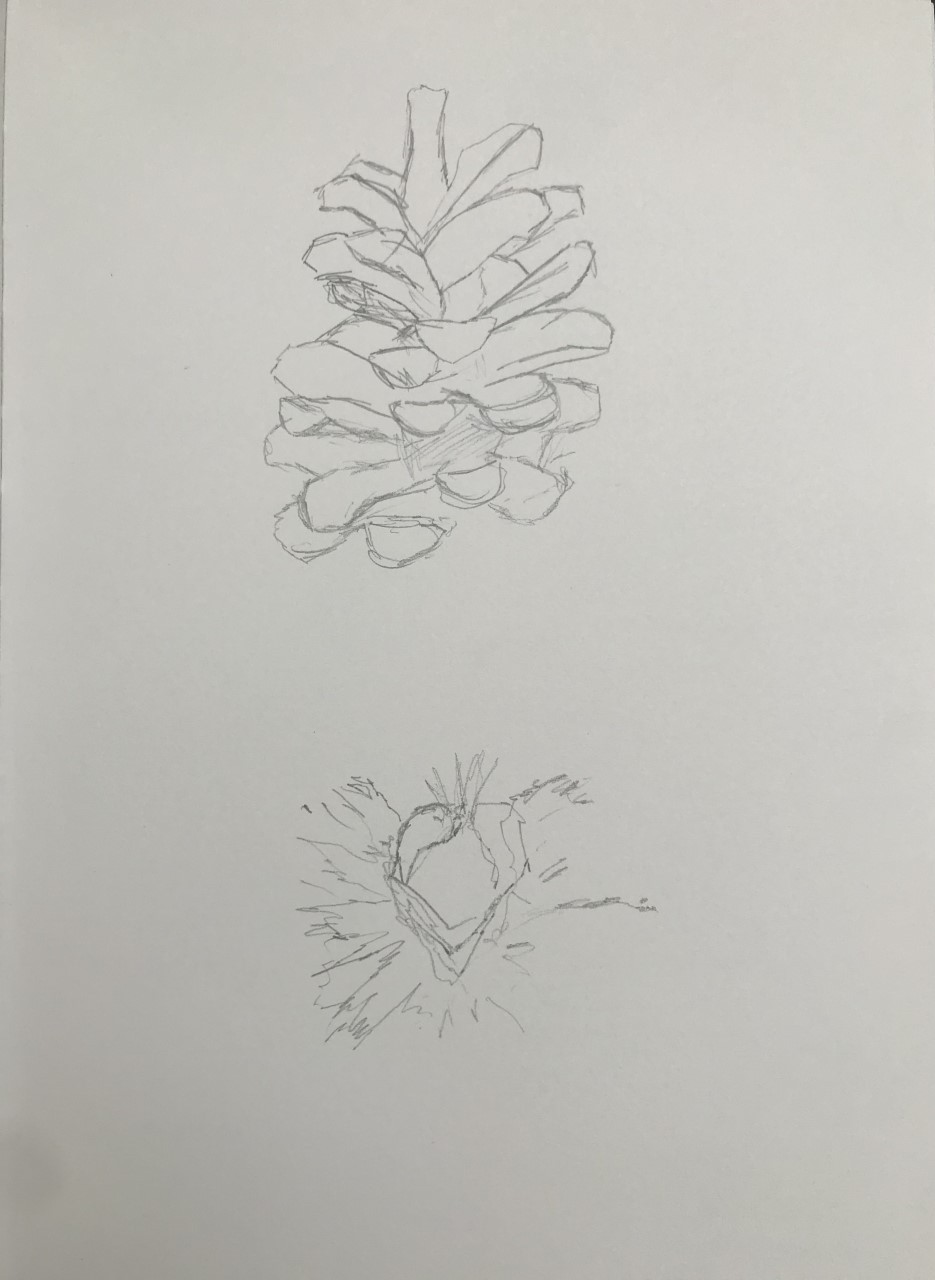On a white piece of sketchbook paper, there are two detailed pencil drawings. The first drawing, positioned at the top middle of the page, is a carefully sketched pinecone. This pinecone features open scales protruding from a central stem, with detailed light shading between the different segments to highlight the pinecone's texture. Below this drawing, near the bottom middle of the page, is a more ambiguous sketch. This second drawing appears to be a rough depiction of a heart, fruit, or possibly a vegetable. It includes a central diamond-like shape from which sharp, electrified lines extend outward. At the top of this object, there is an element resembling a stem or flower, contributing to the uncertainty of its identity. Both sketches are rendered in pencil, displaying varying degrees of detail and shading.